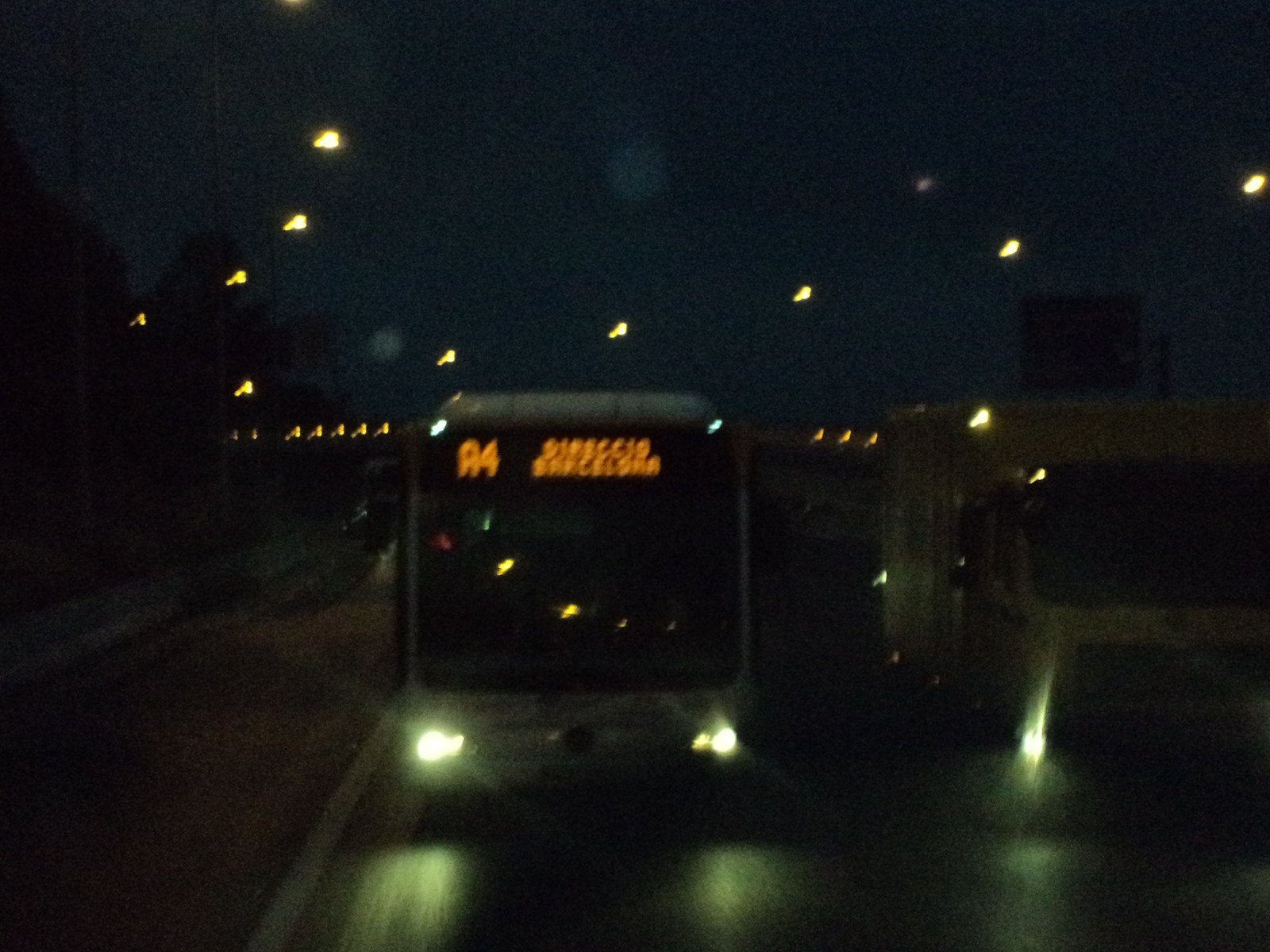The photograph captures a stark nighttime scene with a predominantly dark blue sky, almost black, scattered with around a dozen distant, blurry streetlights. In the lower center of the image, the front of a bus is prominently displayed, illuminated by its bright white headlights. The bus, marked A4, bears an orange, although blurry, electronic display reading "Barcelona" at the front above the windshield, which itself appears dark. Positioned to the right of the bus is a small white truck or van, with some light emanating from it, though its headlights remain off. The vehicles are situated on a road, with a solid white line running along the right side of the bus, and the faint outlines of the street are barely visible. Overall, the image is slightly out of focus, contributing to the mysterious and dimly-lit atmosphere.